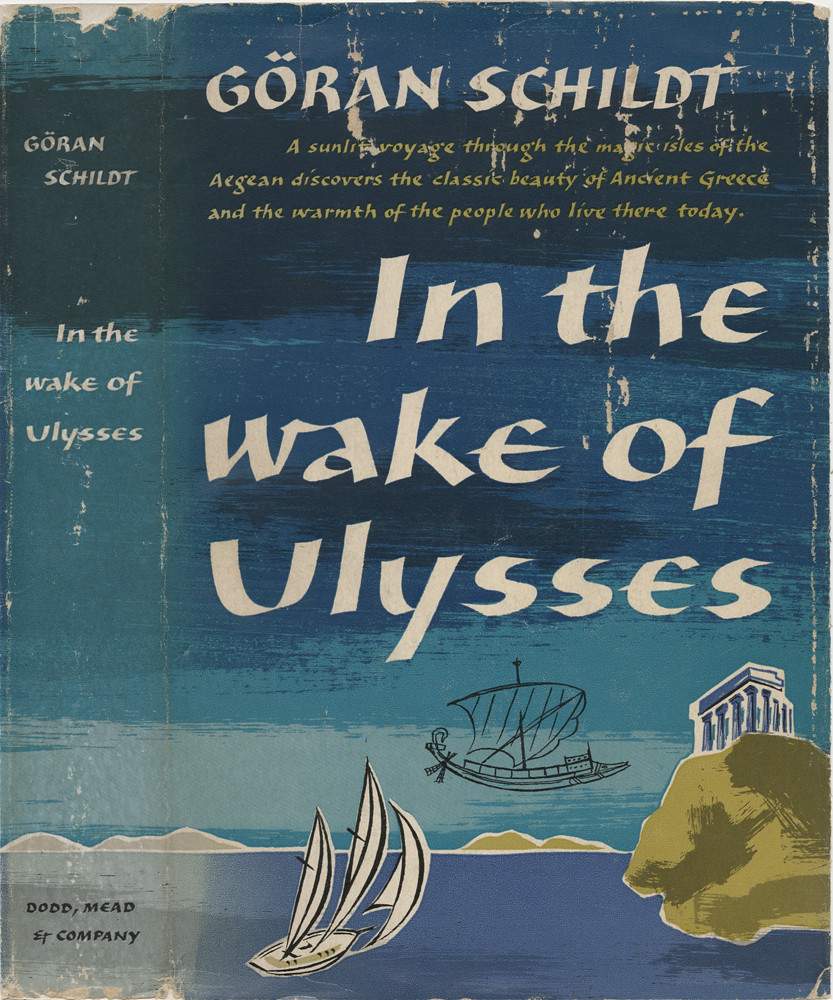The image is of a weathered and vintage book cover titled "In the Wake of Ulysses" by Göran Schildt. The cover features a hand-drawn illustration of a serene sky background with varying shades of blue, transitioning down to a lake and tan mountains. A black and white skiff with three sails sails towards a rocky island adorned with what appears to be remnants of white Roman columns. The book appears to have been folded so that the spine is visible on the front, which also bears the same author name and title in consistent styles. The spine and upper left corner read "Göran Schildt" in white text, and at the very top, the author's name is also repeated. Below his name, in yellow text, it states, "A sunlit voyage through the magic isles of the Aegean discovers the classic beauty of ancient Greece and the warmth of the people who live there today." At the bottom of the cover, the publisher's name, "Dodd, Mead, and Company," is printed in black. The cover shows significant wear, with creases and peeling at the edges, underscoring its vintage nature.